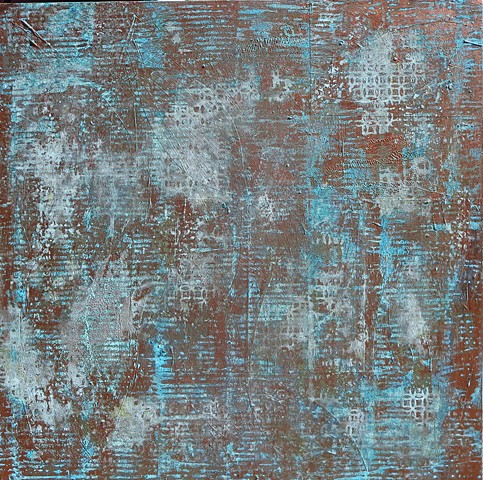This image depicts a piece of abstract artwork characterized by a brown-red, burgundy-like background, suggesting a textured or ribbed surface, perhaps akin to a canvas or a wall. Superimposed on this reddish-brown backdrop are various shades of light blue and white paint, applied in an irregular manner. The blue seems to be applied with a roller, creating vertical textures, while the white paint includes both random splotches and stenciled patterns resembling caning. The overall effect is one of layered remnants, as if previous materials were removed, leaving behind a multi-faceted, textured composition. This combination of colors and techniques contributes to a dynamic and thought-provoking visual experience.